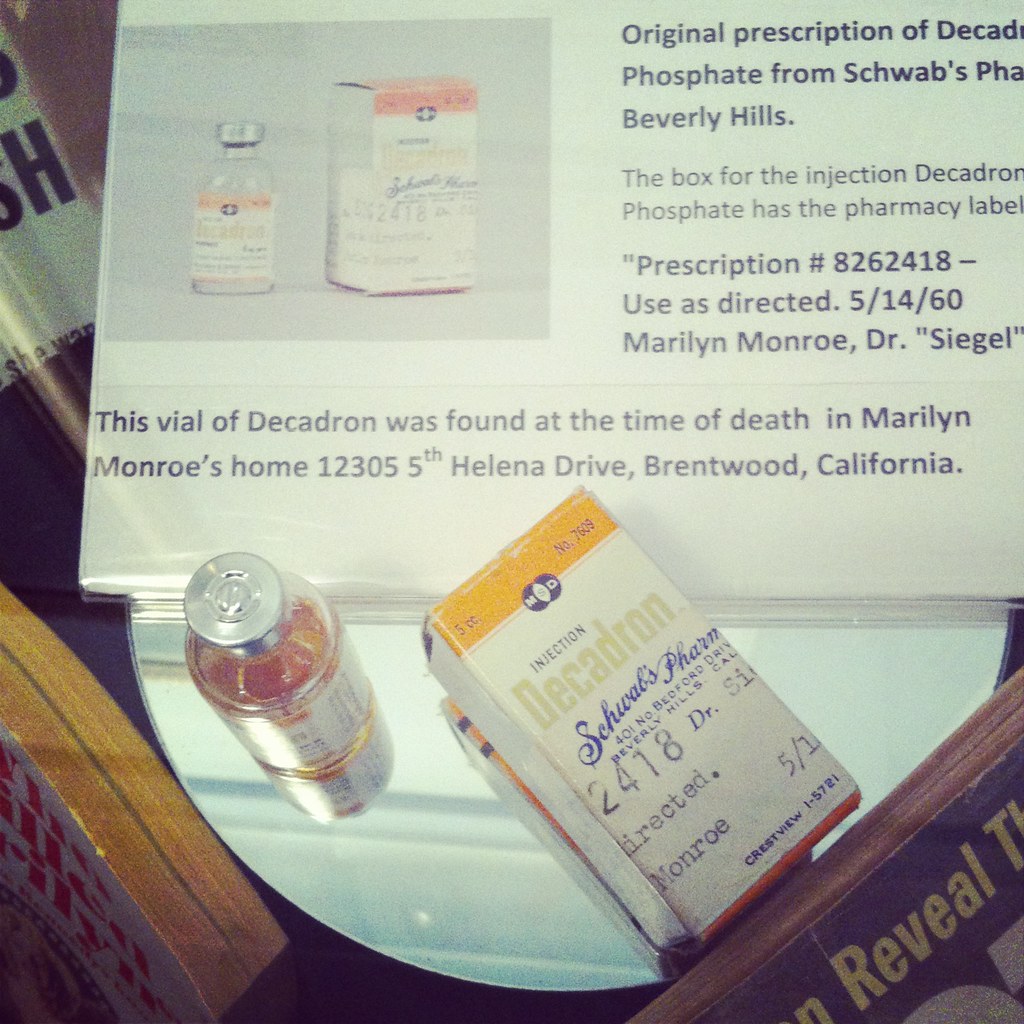This image depicts a highly detailed museum exhibit centered around a historic prescription from Schwab's Pharmacy in Beverly Hills, featuring objects tied to Marilyn Monroe. At the bottom left corner, there is a book, while at the bottom right corner, another book corner is visible, emphasizing the exhibit's literary context. In the center, resting on a table, lies a white box labeled "Injection Decadron." Next to it, the actual medication is contained in a vintage glass vial. Prominently displayed near the top of the image, an informational sign reads "Original Prescription of Decades Phosphate from Schwab's Pharmacy, Beverly Hills" and includes historical data such as a prescription number and the year 1960, along with Monroe's address in Brentwood, California. This setup, likely part of an indoor museum exhibit, provides a glimpse into the late actress's life, complete with the prescription found at her death. The array of colors, including yellow, red, white, light blue, orange, black, and white, adds to the visual richness of the exhibit.